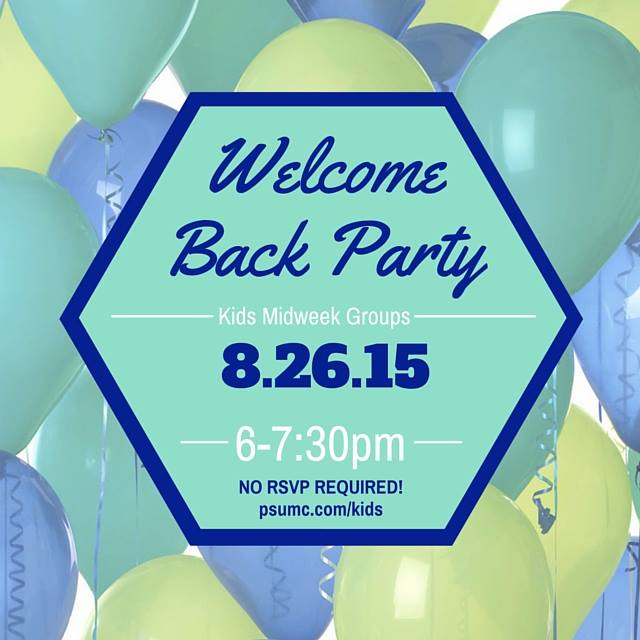This image features an invitation decorated with an array of balloons in varying shades of green and blue, accompanied by their festive curly strings. At the center of this vibrant background is a hexagon-shaped sign, which has a light green interior and a bold dark blue border. At the top of the hexagon, in a deep blue cursive font, it reads "Welcome Back Party." Below this, in smaller white text, it announces "Kids Midweek Groups" followed by the event date in large bold dark blue numbers: "8.26.15," indicating August 26, 2015. The time for the event, "6-7:30 p.m.," is listed beneath the date in white text. At the bottom of the hexagon, it states, "No RSVP required," with a web address, "psumc.com/kids," suggesting that the event is organized by the United Methodist Church for children's groups.